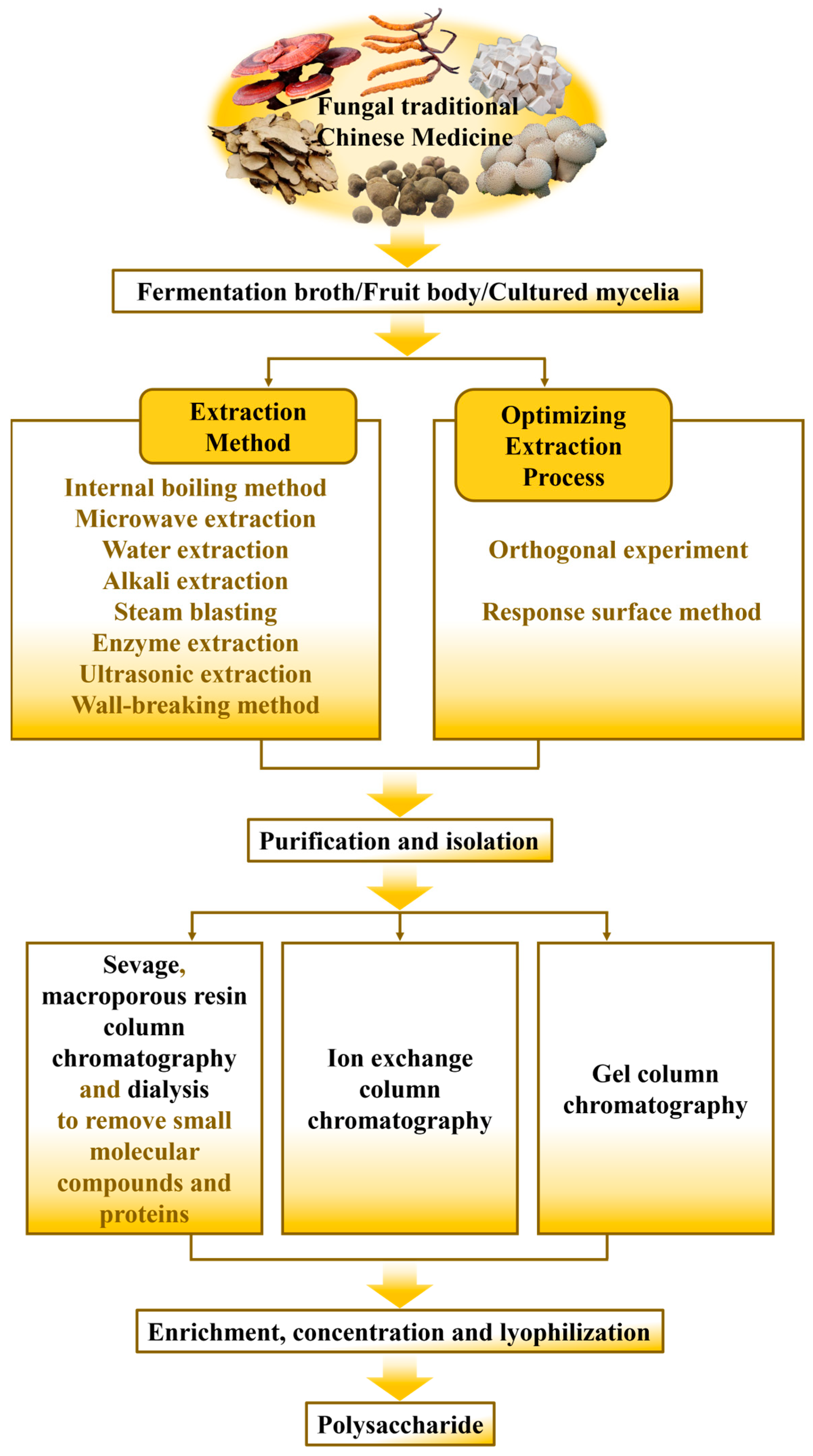This detailed infographic illustrates the process of creating fungal traditional Chinese medicine. At the top, within a yellow oval, are images of six different Chinese medicinal herbs, with the title "Fungal Traditional Chinese Medicine" prominently displayed in black text. A yellow arrow descends to the next stage, which lists "Fermentation Broth," "Fruit Body," and "Cultured Mycelia." This arrow leads to two branching boxes labeled "Extraction Method" and "Optimizing Extraction Process," each filled with brown explanatory text. The top of each box is white, transitioning to a yellow gradient at the bottom.

These two boxes connect via arrows to another rectangular section labeled "Purification and Isolation." From here, the flowchart branches into three separate boxes titled "Savage Macroporous Resin Column Chromatography and Dialysis," "Ion Exchange Column Chromatography," and "Gel Column Chromatography." A subsequent yellow arrow points to another process phase labeled "Enrichment, Concentration, and Lyophilization," which finally leads to a box that reads "Polysaccharide." The overall design features a dominant yellow theme and follows a linear, top-to-bottom flowchart format with clear educational intent.